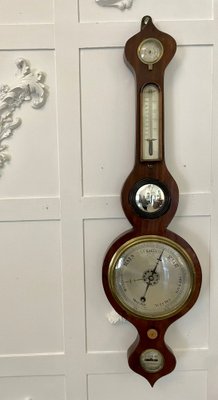The image depicts an old-fashioned banjo barometer made of dark brown wood, hanging vertically on a white paneled wall with a raised grid pattern and filigree decorations. This wooden instrument comprises three distinct compartments: a thermometer located in the neck, a larger barometer face near the bottom with an arrow pointing northeast, and possibly a hydrometer. The topmost and bottommost sections feature small circular dials, though the low resolution of the photograph obscures their details. The wall behind the device is devoid of any other objects or text, highlighting the contrast between the ornate instrument and its simple backdrop.